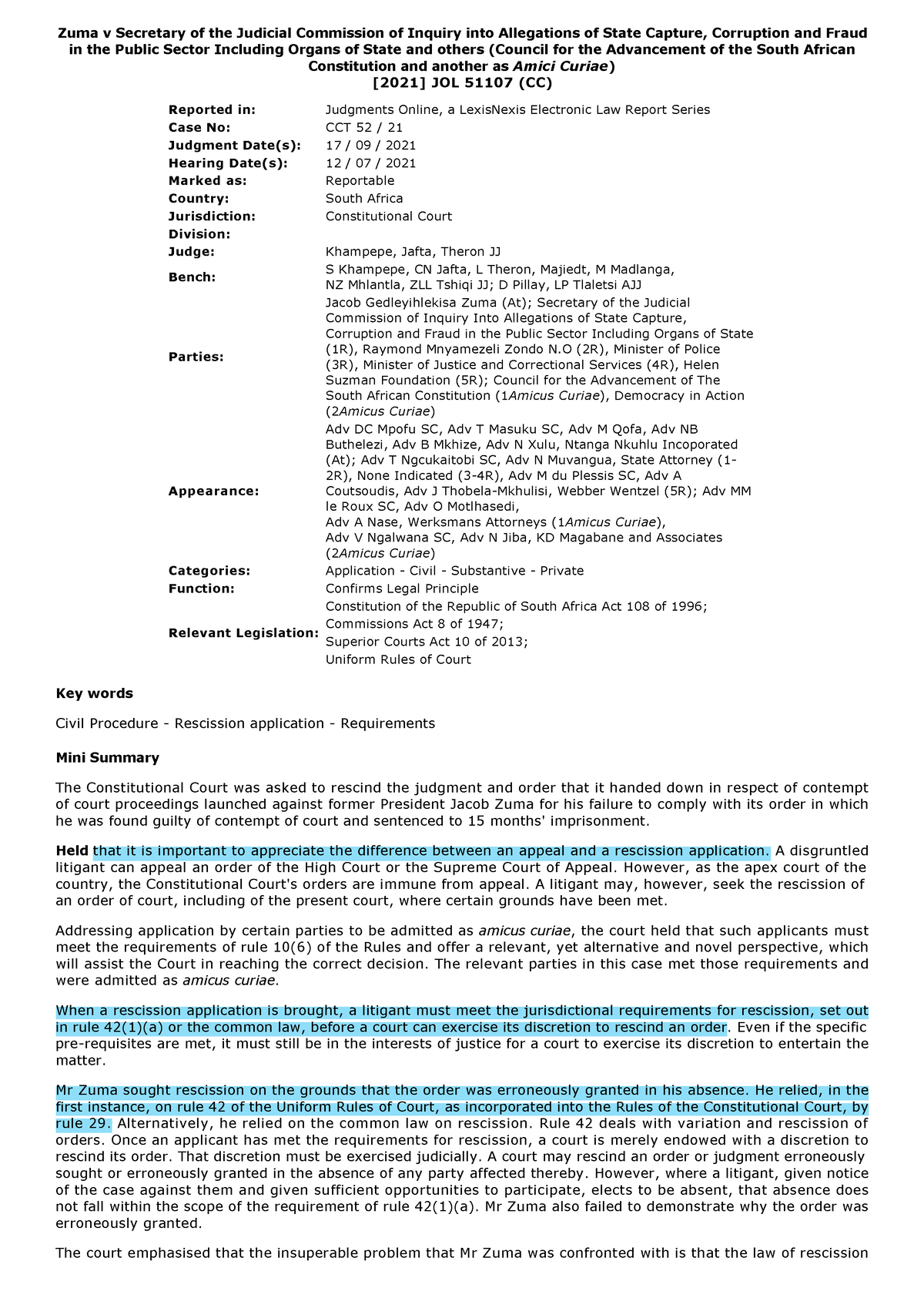Image Description: The image appears to be a document, likely an email or a summary of information, with text that is primarily illegible due to its small size. At the top, a fragment of the title can be discerned, potentially stating, "The Z Versus V Secretary of the Judicial Commission of Inquiry into Allegations of State Capture, Corruption, and Fraud in the Public Sector, Including Organs of State and Others." 

Additionally, there is a mention of "People for the Advancement of the South African Constitution," followed by incomplete or unclear text. Beneath this heading, the document contains approximately five short paragraphs of text. Above these paragraphs, a few bullet points are visible. However, the specifics of these bullet points and paragraphs remain indecipherable. No other distinguishing details or information can be extracted from the image.